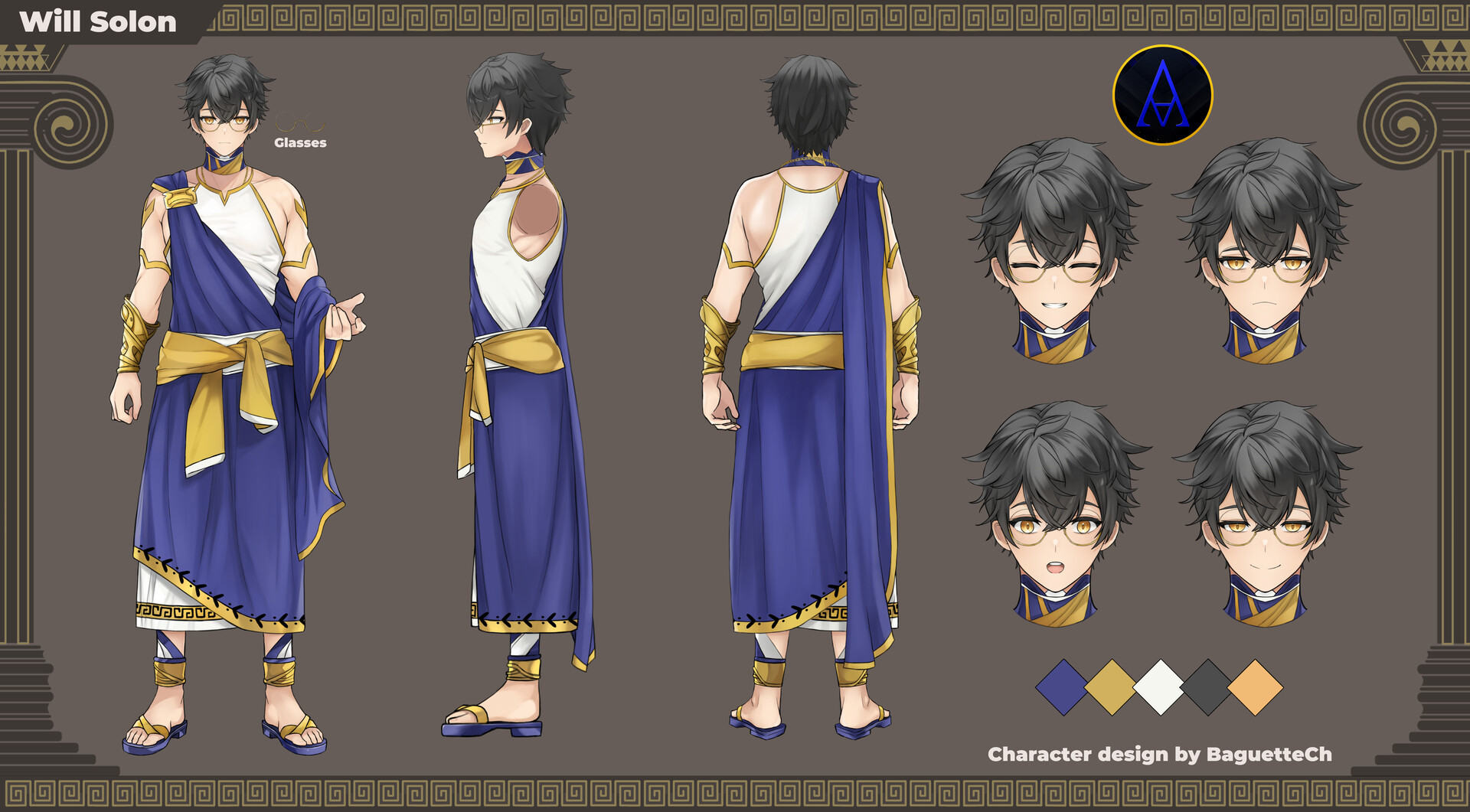The image depicts an animated character named Will Solon, designed by Van Gweddich (or Baguette CH). Will Solon is a small Asian man with wispy black hair and glasses. He is wearing an outfit that resembles Roman attire, consisting of a white and purplish-blue robe tied at the waist with a gold sash, and purple and gold sandals. He also has gold accessories around his arm. The character is shown in three different angles: front, side, and back, providing a comprehensive view of his attire. To the right of these images, there are four headshots displaying different facial expressions (laughing, sullen, surprised, and happy). The background is brown with pillars, and the top of the screen displays the name "Will Solon." Various colored diamonds (blue, gold, white, black, beige) are positioned at the bottom.